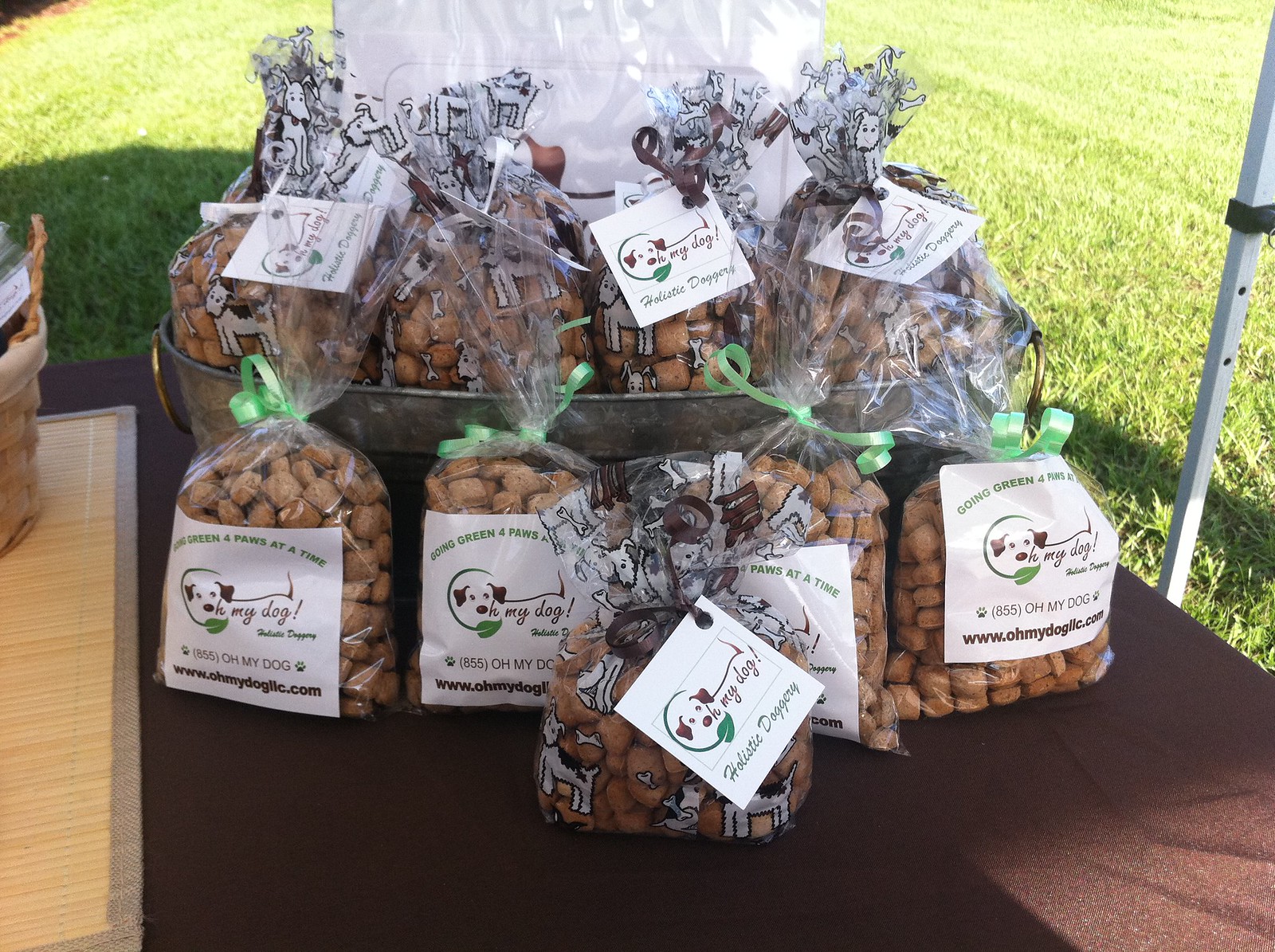In this photograph of an outdoor market, a prominent display of specialized dog treats captures the focus. The scene is set on a bright, sunny day with a lush, green grassy backdrop. The market stall is shaded by an umbrella or awning, with visible supporting poles indicating overhead cover.

The main feature consists of numerous translucent cellophane bags filled with brown dog treats. These bags are elegantly tied with light green ribbons, appearing almost like gift bags. Each bag has a label that reads "O My Dog" or "Oh My Dog," with a logo featuring a Dachshund-like dog whose body forms part of the lettering. The label is adorned with additional text, including "Holistic Doggery" in blue and the slogan "Going Green Four Paws at a Time" in green. A website, www.omydogLLC.com, and phone number, 885-OMYDOG, along with two black paw prints, are also printed on the label.

The bags are arranged in two main groupings: some are neatly placed on a brown tablecloth-covered table while others are contained within a large, silver-colored metal tub that resembles a bathtub and features gold handles. Adjacent to the main table is another table, only partially visible, displaying a brown wicker basket.

This well-organized display suggests a thoughtfully curated market booth dedicated to promoting and selling eco-friendly, holistic dog treats.